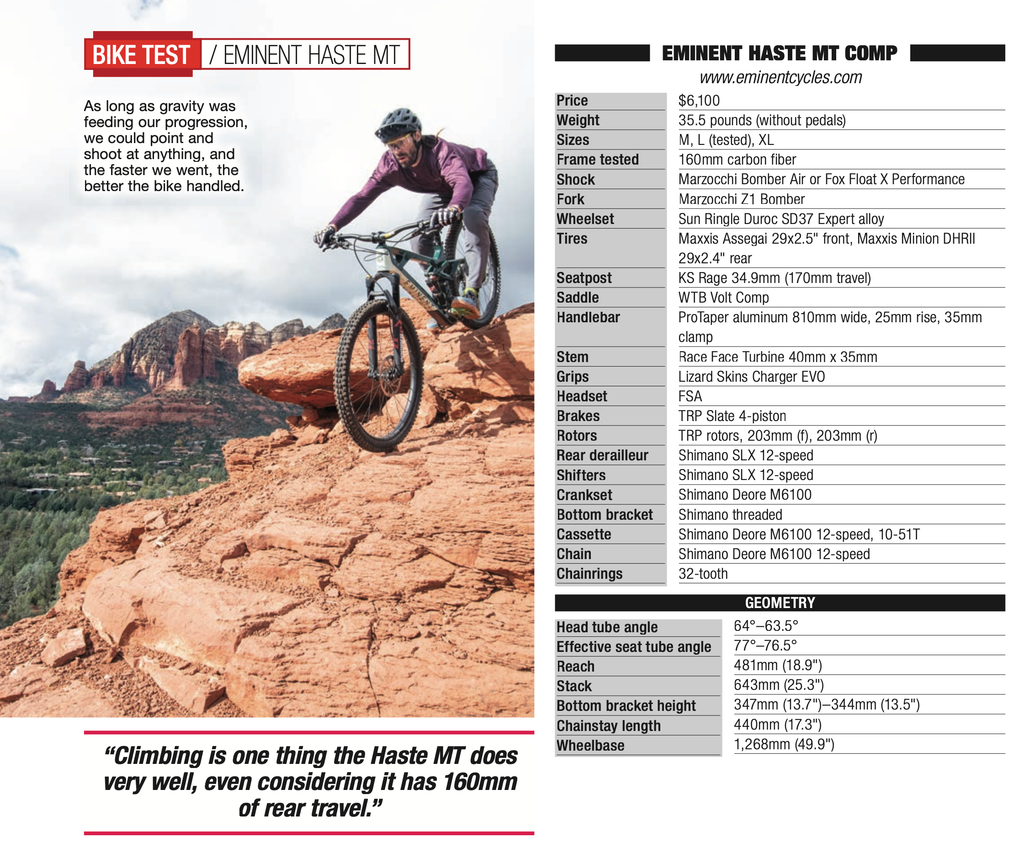The image features a dynamic scene of a man in a purple long-sleeve shirt and dark gray helmet, riding a mountain bike down a steep, clay-colored canyon rock. He is positioned standing on the pedals with his weight shifted to the back of the bike, which sports a white bottom and blue top. This dramatic descent is set against an overcast sky with gray clouds and a grassy background, highlighting the rugged terrain.

To the left, there's a photograph headed by a red banner with white text stating, "Bike Test: Eminent HAST-MT." Below, a paragraph reads, "As long as gravity was feeding our progression, we could point and shoot at anything, and the faster we went, the better the bike handled." Further down, another caption states, "Climbing is one thing that HAST-MT does very well, even considering it has 160 millimeters of rear travel."

To the right of the image, the specifications for the bike are listed, including the model, "Eminent HAST-MT Comp," along with details such as the price ($6,100), weight (35.5 pounds without pedals), available sizes (M/L as tested and XL), and key components. The bike's shocks are specified as either Marzocchi Bomber Air or Fox Float X Performance, the fork as Marzocchi Z1 Bomber, and the wheelset as Sun Ringle Düroc SD37 Expert Alloy. The overall presentation emphasizes both the bike's technical capabilities and its performance under extreme conditions.